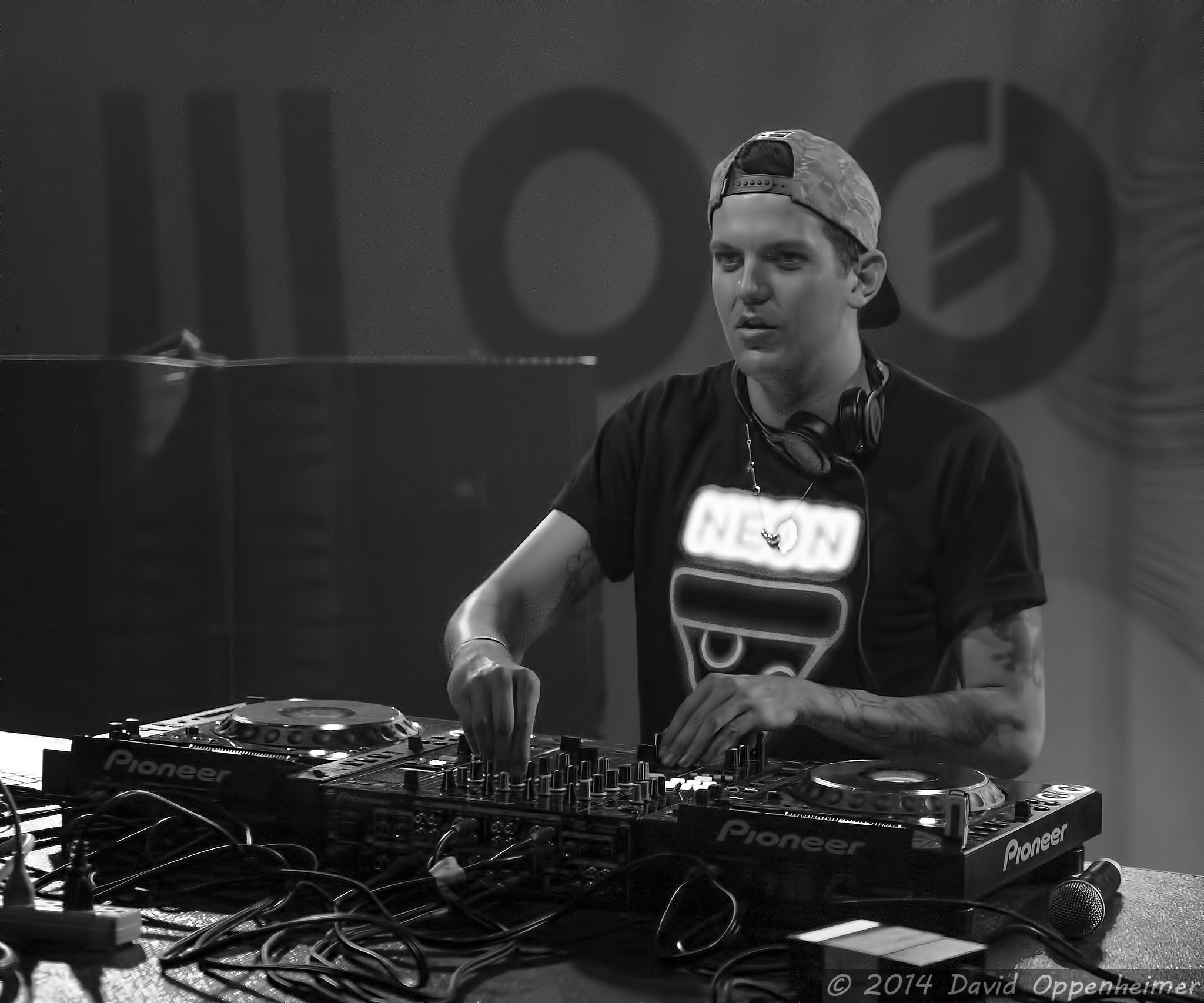The image showcases a DJ spinning discs, centrally positioned against a gray, black, and white background. The DJ, wearing a backward hat, gazes slightly to the left while adjusting knobs on his Pioneer DJ mixer. The foreground reveals a cluttered table with numerous cables and plugs connected to a surge protector, emphasizing the intricate setup. A microphone rests beside the mixer on the table. The backdrop is decorated with three vertical lines and two unique O's, one featuring a diagonal backward C. Notably, the image is marked with the text "2014, David Oppenheimer" in the bottom right corner, establishing the copyright and adding to the overall layout. The indoor setting, likely a club, contributes to the professional and immersive atmosphere of the scene.